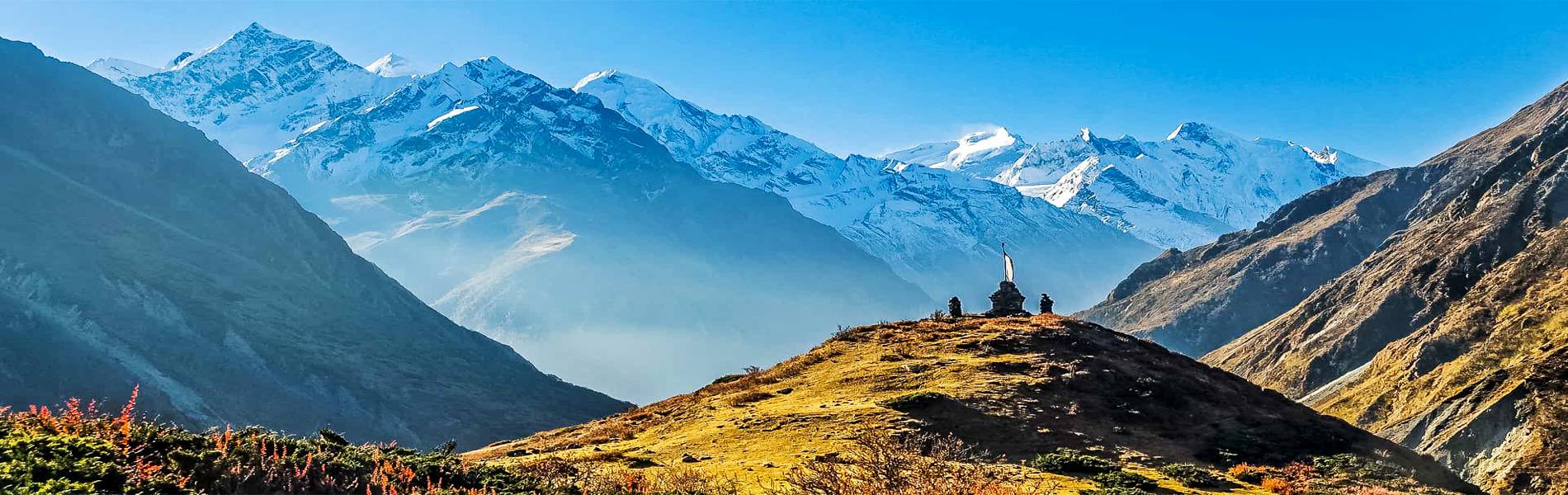This wide-angle, rectangular outdoor photograph captures a striking mountainous landscape during the daytime. In the foreground, on the left-hand side, we see a grassy hill with patches of red foliage, which rises towards the center before sloping down to the lower right corner. At the top of this hill, there are three rock cairns, the largest of which features a white flag. Surrounding this hill and extending into the mid-ground are mountainsides bathed in golden hues, with one particularly steep and shadowed slope on the left, cast in gray tones. In the background, the majestic snow-capped peaks of what appears to be the Himalayan mountain range stretch towards a clear, blue sky. The serene and expansive scene is highlighted by the contrasting colors and elements of nature, suggesting the purity and grandeur of a high-altitude landscape.